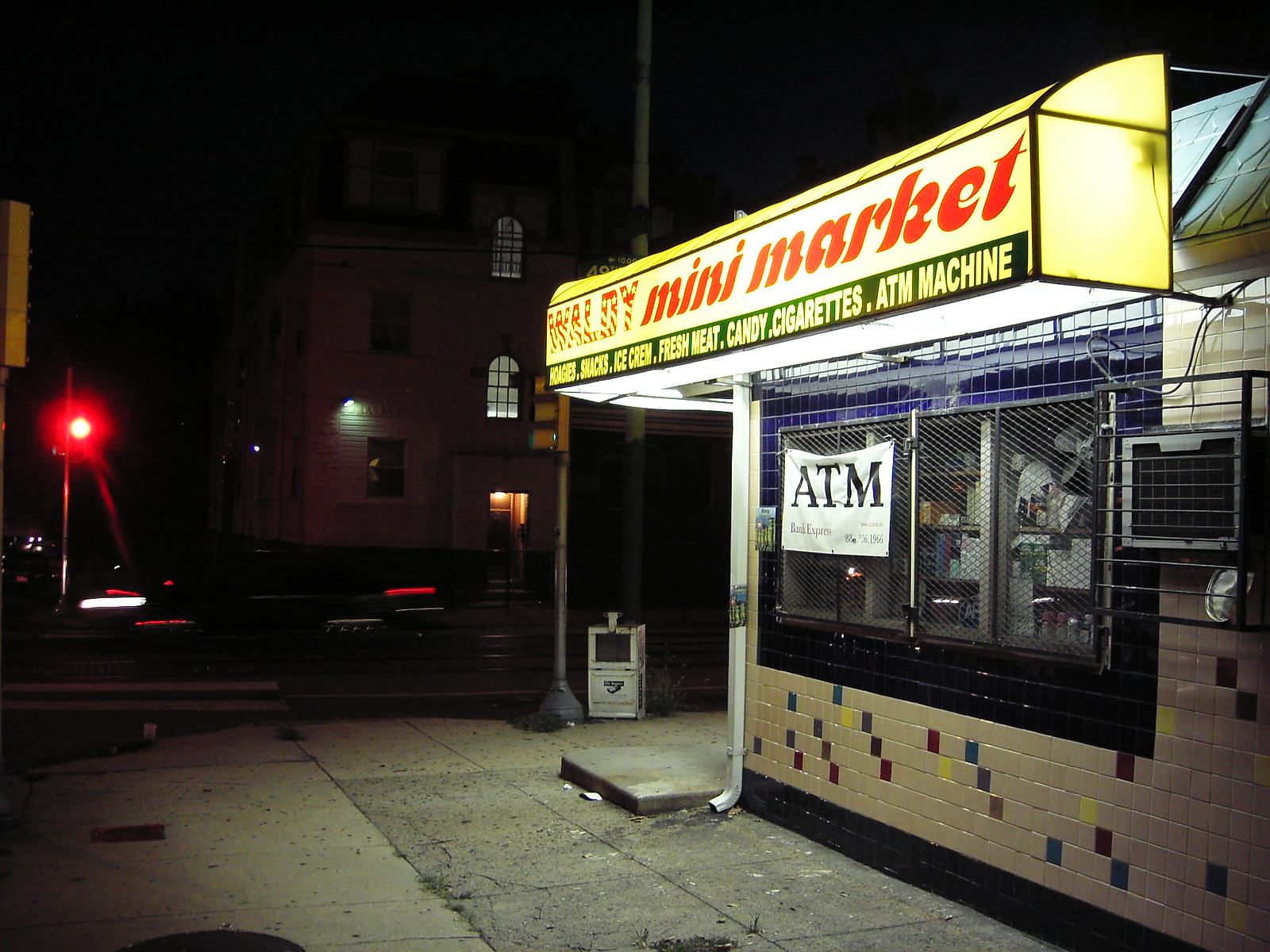The photograph captures a nighttime scene at the corner of a street in a city, centered on a convenience store named Waldie Mini Market. The store, located on the right-hand side, features a distinctive beige exterior adorned with randomly placed blue, red, yellow, and brown tiles. An illuminated awning, prominently marked "Waldie W-A-L-D-Y Mini Market" in red, also lists available items such as snacks, ice cream, fresh meats, candy, cigarettes, and ATM services. The front of the store includes a cage-covered window with a banner advertising an ATM, a window unit air conditioner also shielded by a cage, and a sidewalk littered with a few pieces of trash. The sidewalk leads up to the store entrance, marked by a white tile foundation interspersed with colorful tiles. Nearby, a newspaper box sits empty, suggesting it is late at night as no people are present in the scene. Across the street, multi-story buildings loom in the background, and a red stoplight glows on the left side of the frame. A few cars are visible driving in the distance, adding to the quiet, late-night atmosphere of this urban corner.